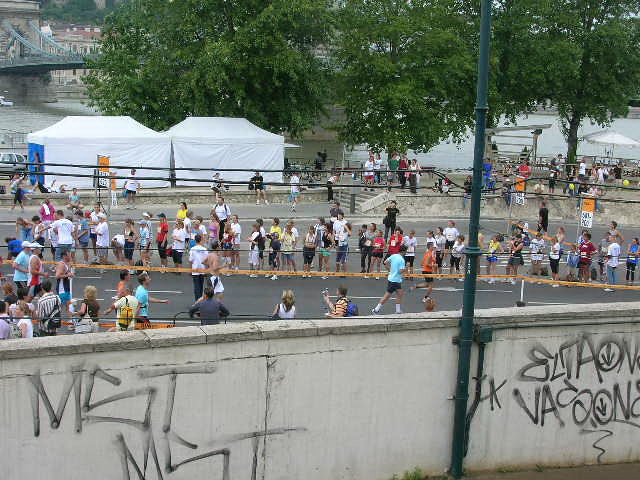This photograph, likely taken from the second floor of a building or a rooftop, captures a marathon event on a city street. A concrete retainer wall with graffiti and a dark blue metallic pole defines the foreground. Beyond the wall, the street, running left to right, is lined with roped-off lanes for marathon runners, surrounded by spectators who stand and sit on either side. Two white tents, presumably for the event participants, are set up on the right side of the road. In the background, there's a park area with large trees and a waterway spanned by a distant bridge. The scene is bathed in gray tones, reflecting the urban setting and overcast weather, suggesting a typical city marathon atmosphere.